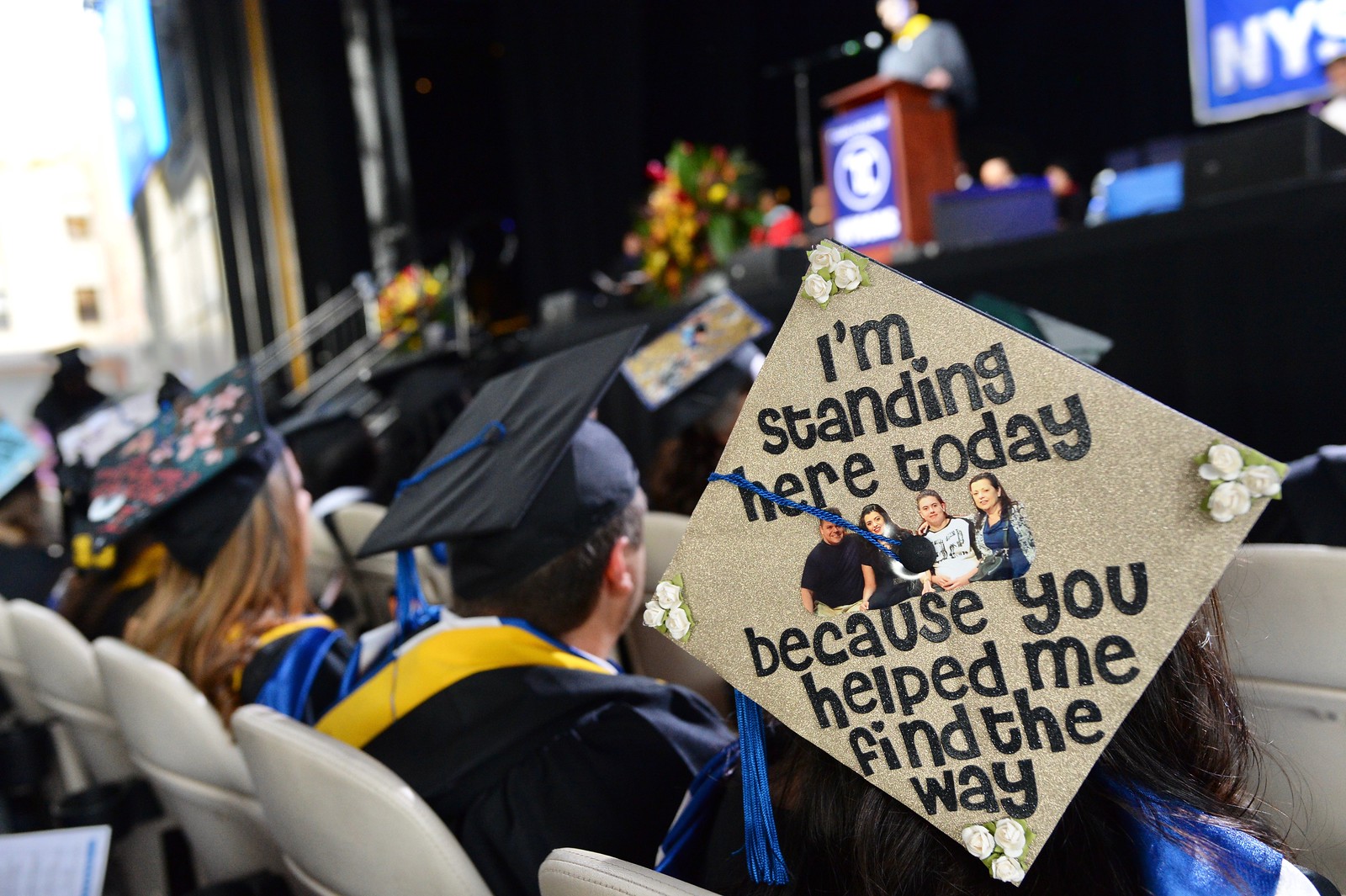The image captures a vibrant graduation ceremony, with a view down an aisle leading to a stage. The scene is somewhat blurry in the background, but you can make out a speaker standing at a wooden podium draped with a purple cloth. In the upper right-hand corner, a sign reads "NYS" or possibly just "S," hinting that this could be a New York college. The attendees are seated with their backs to the viewer, gazing at the stage. At the forefront, there's a young woman with blonde hair, adorned in a graduation gown and cap, seated beside a man with short dark hair, also in a gown. Notably, the woman's cap is vividly decorated with a heartfelt message: "I'm standing here today because you helped me find the way," accompanied by pictures and flowers at each corner. Her cap features gold paint or glitter accentuating the letters. In contrast, the man next to her wears a plain cap with a blue tassel. Although slightly obscured, another young woman a few seats away also has a message on her cap. The stage, primarily black with blue and yellow decor, reflects the somber yet celebratory atmosphere of this momentous occasion. Daylight streams in from the left, adding an extra touch of brightness to the scene.